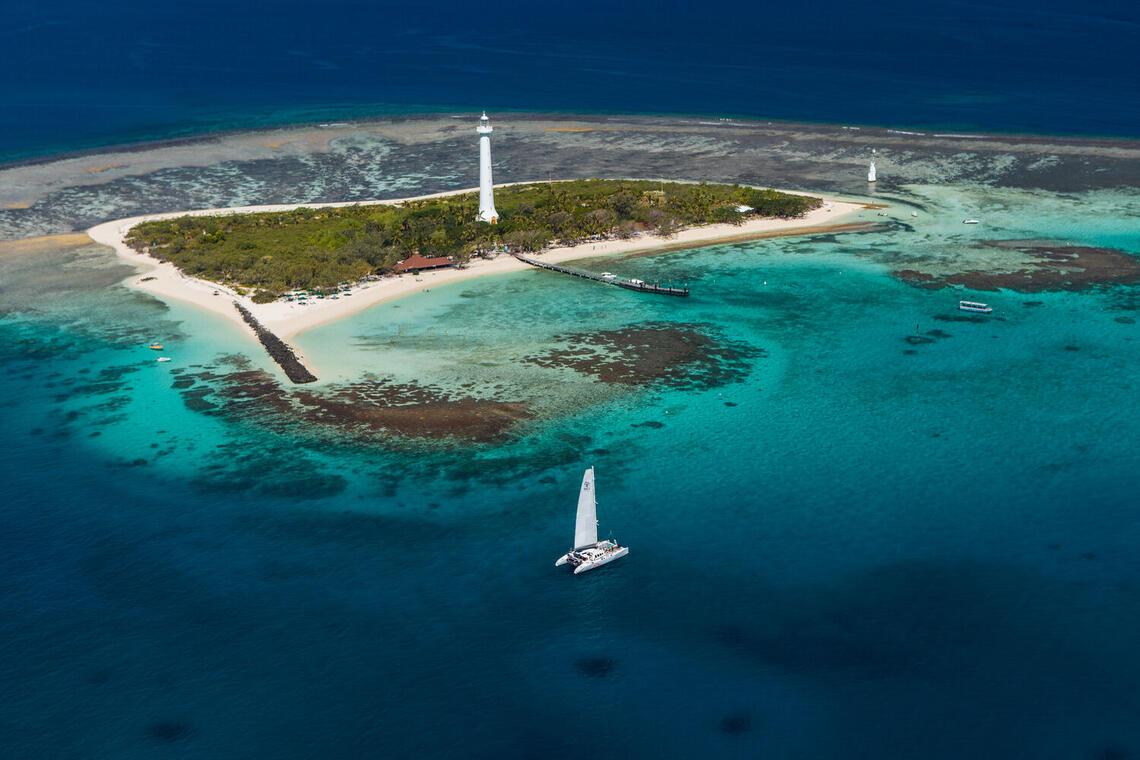In this breathtaking aerial photograph, a pristine island is the focal point amid the vast, dark blue ocean that gradually turns to lighter hues as it nears the shore. The island is encircled by dazzling white sand beaches, and at its center stands a towering, white lighthouse. Stretching out from the lighthouse, a large dock extends into the ocean, leading to a pontoon boat and a sailboat with a giant white sail approaching the island's coast. The crystal-clear water reveals shades of green and brown coral as well as smaller submerged islands. Lush greenery blankets the island, peppered with grass and a few trees. There are also small structures and green umbrellas visible on the beach. In the top right corner, another smaller lighthouse can be seen standing in the water against the backdrop of an expansive sky.